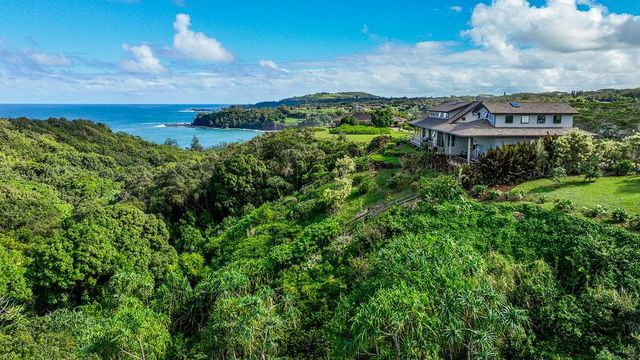This is a detailed landscape photo of a picturesque, remote location on a Hawaiian island. The focal point is a substantial two-story house with white walls and a dark brown roof, sculpted into an L-shape. The house boasts a small front porch and sits elevated on a hillside, overlooking the stunning blue ocean to the upper left. Beautifully set against a backdrop of a clear blue sky adorned with fluffy white clouds, the house is reached by a walkway or steps leading up the slope. This idyllic setting is surrounded by an abundance of tropical plants and trees, which blanket the undulating terrain in a vivid array of green hues. Clusters of bright green trees intermingle with darker foliage, adding depth to the landscape. Additional houses dot the distant background in this lush, hilly expanse, enhancing the remote charm of the location. The foreground features grassy areas on both the right and left, seamlessly blending into the vibrant natural scenery.